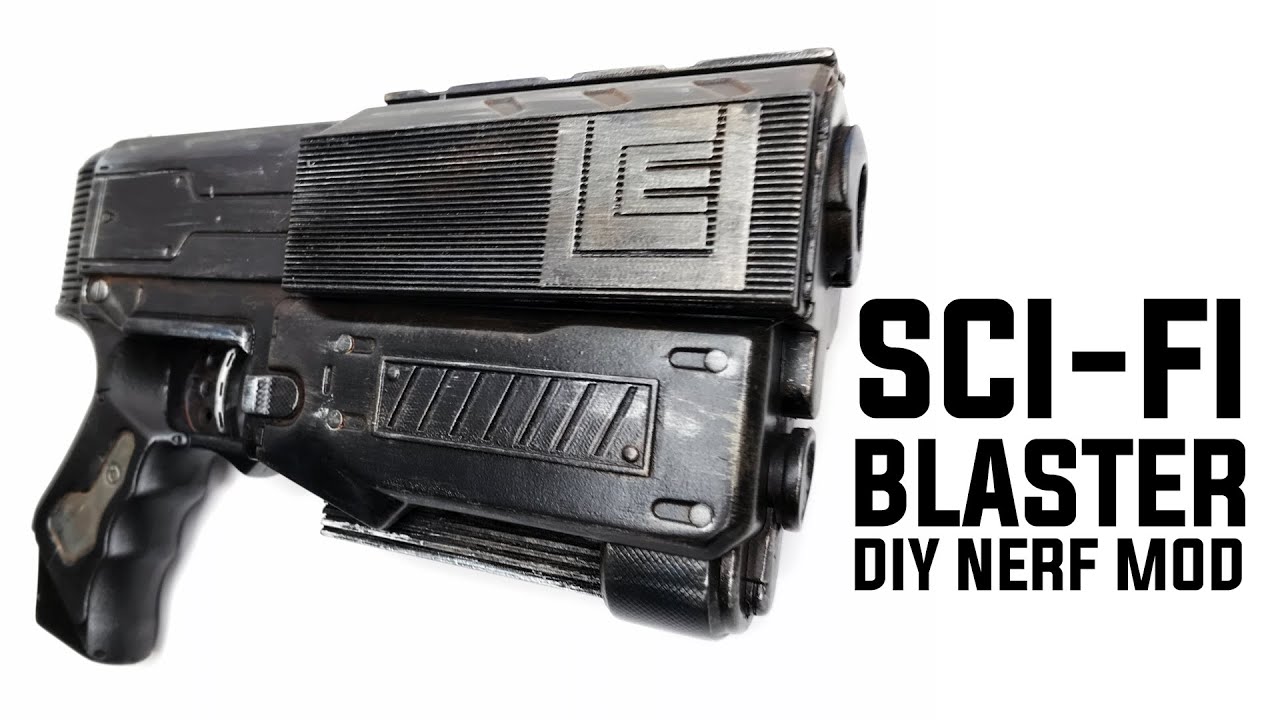This advertisement features a landscape-oriented, black-and-white photograph of a modified Nerf gun. The gun, appearing highly realistic, is primarily black with gray details and has an overall scuffed-up look that gives it the aesthetic of a well-used sci-fi blaster. Positioned horizontally in a side profile, the gun’s grip is on the left side of the image, and it points to the right. The barrel is notably tall and features a black rectangle on top, adorned with a chrome emblem that seems to depict embedded letters like U-C-E. Below this emblem is a black rectangular cartridge with a barrel shape. Etched on the side of the gun is the letter "E," adding to its detailed design. On the right-hand side of the image, black text reads "Sci-Fi Blaster," with the subtitle “DIY Nerf Mod” underneath in smaller print. The plain white background makes the gun appear as if it is floating, enhancing the advertisement’s clean and focused presentation. This sophisticated mock-up effectively merges graphic design with photography to emphasize the gun’s sleek and realistic transformation from an original multi-colored Nerf toy to a sophisticated sci-fi weapon.